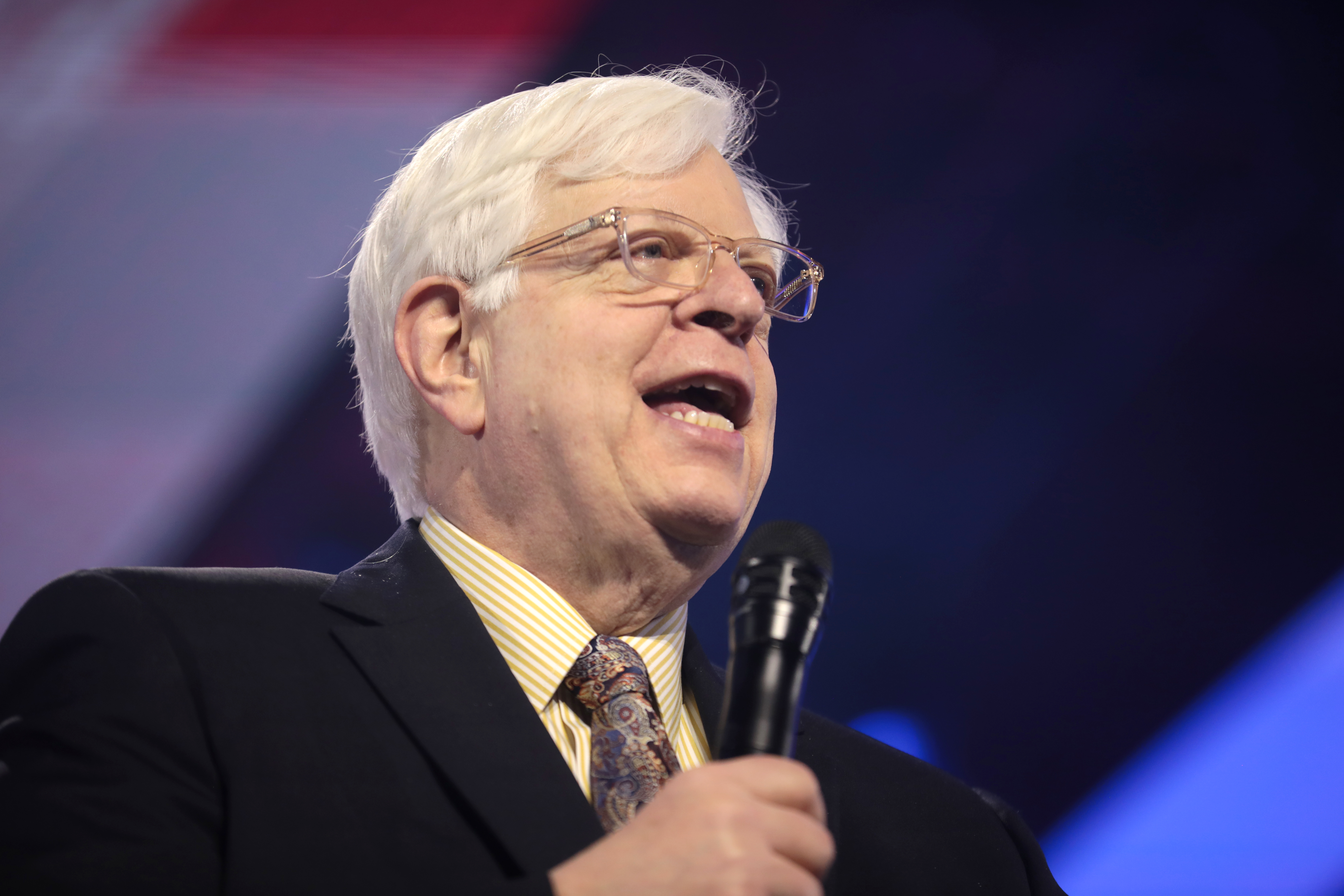An elderly man, likely in his late 60s or 70s, stands at the center of the photograph, holding a black microphone close to his mouth. He has white hair and wears clear glasses, adding to his distinguished appearance. Clad in a black suit jacket, he pairs it with a white and yellow-striped shirt and a vividly colorful tie, showcasing a splash of personality. The background is deliberately blurred, featuring an array of lights or a screen with gradients of blue at the bottom and transitioning into white and red hues towards the top. This vibrant backdrop adds depth to the image while keeping the focus on the man, who appears to be engaged in speaking, possibly giving a presentation or delivering a speech. Despite his commanding presence, his identity remains unknown.